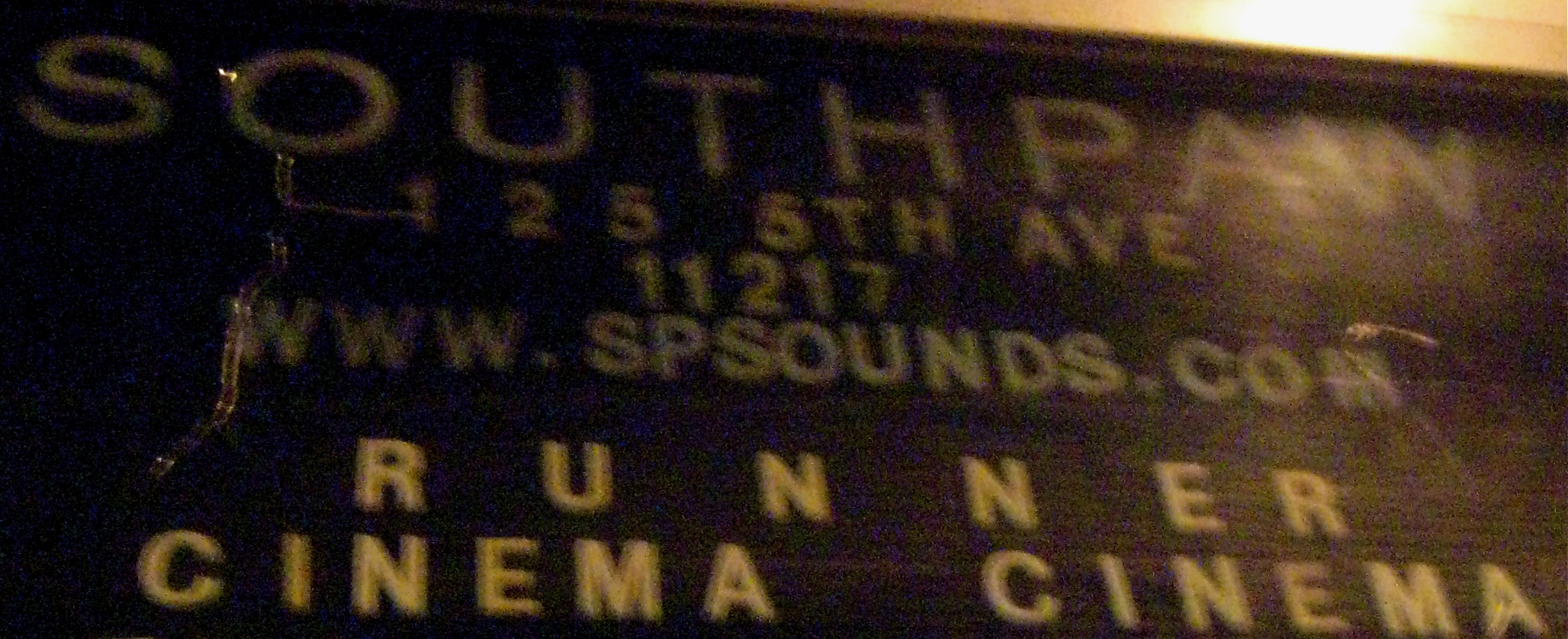In this somewhat grainy and dimly lit close-up photograph, a black marquee sign occupies the frame. At the top of the sign, large white capital letters prominently display the word "Southpaw." Below this, the street address "125 5th Avenue, 11217" is partially visible, with the numbers and some letters cloaked in shadow. Further down, the website address "www.spsounds.com" is inscribed but similarly obscured by darkness. Underneath the web address, the word "runner" appears, followed by the repeated word "cinema," with noticeable spacing between the two instances. A bright light affixed above the sign casts illumination sporadically, accentuating the letters "paw" in "Southpaw" and the lower lines of text, while leaving the words "South," the majority of the address, and part of the website shrouded in shadow.